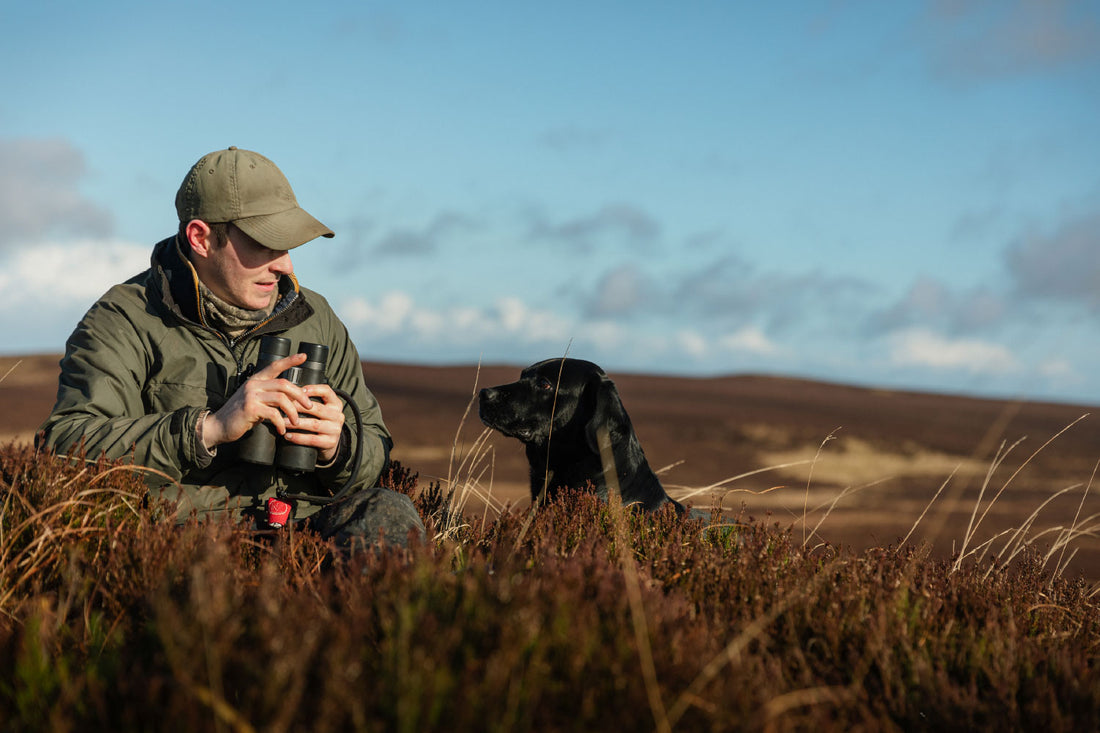This photograph captures a serene outdoor scene featuring a middle-aged man and his black retriever dog, likely engaged in hunting or bird-watching activities. Set in a vast, open field devoid of buildings or other people, the setting is characterized by the brown, wintry grass that adds a rustic charm. In the foreground, tufts of dark brown and beige, wheat-like grasses frame the subjects. The man, seated on the left side of the frame, is attired in hunter gear that includes a dark green jacket, olive green cap, and a camo face cover pulled down under his chin. He firmly grips a pair of large black binoculars with both hands, directing his gaze downward and to the right at the dog. The dog, slightly behind the grass, showcases a thick neck and medium-length black fur, looking attentively to the left at the man, perhaps awaiting a command. The background of the image is dominated by a pale blue sky, scattered with dark gray and white puffy clouds, while the distant horizon reveals deep brown land interspersed with beige patches, creating a peaceful and immersive natural environment.